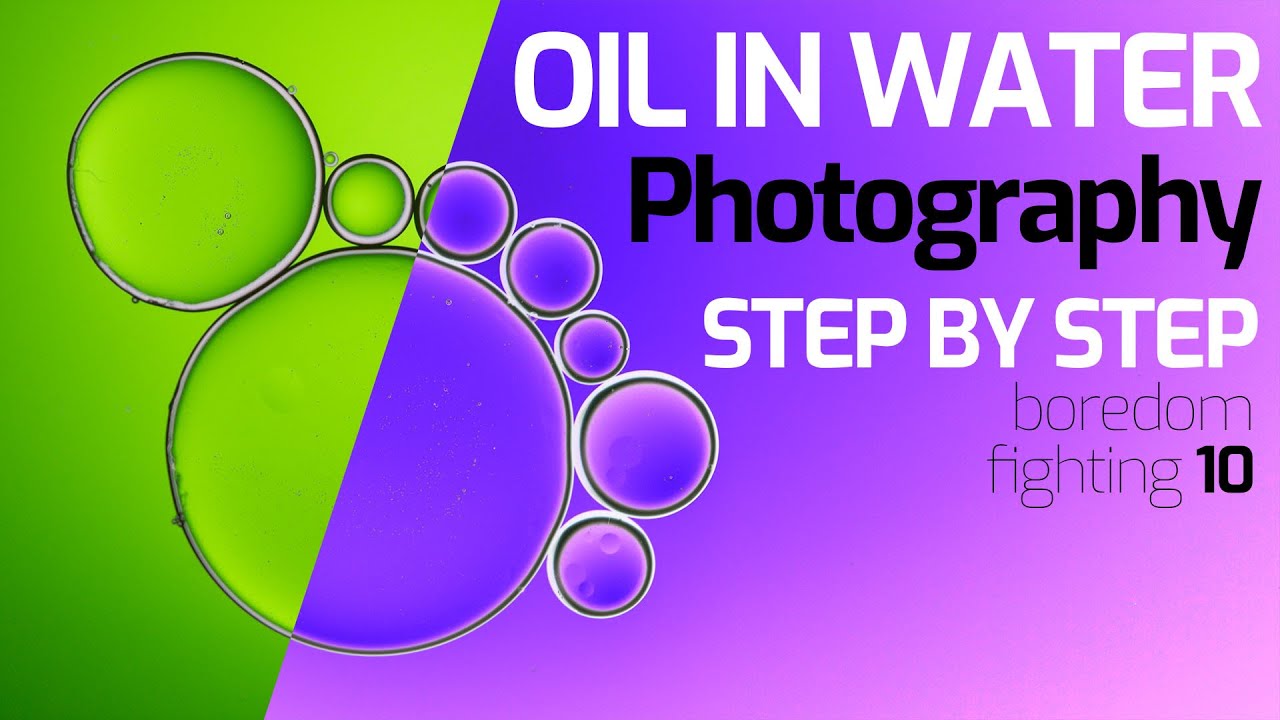This digital graphic design, possibly created in Photoshop, showcases a striking blend of colors and textures. Dominated by a purple and blue gradient covering most of the image, the design transitions sharply into a chartreuse green and yellow-green gradient on the left, starting at the first fourth of the image and separated by a diagonal line. Central to the composition is a large bubble, half green and half purple, suggesting an oil drop. This bubble is adorned with a ring of smaller bubbles of varying sizes, spanning from the 11 o'clock to the 4 o'clock position, creating a dynamic overlap across the purple and green sections. The text elements are prominently placed on the right side, with large block white text reading "Oil and Water," followed by black text "Photography" slightly below. Underneath, in slightly smaller white text, it reads "Step-by-Step," and then "Boredom Fighting" in very thin black text, culminating with a bold "10." This composition combines vibrant colors and a playful arrangement of bubbles to create a visually engaging piece.